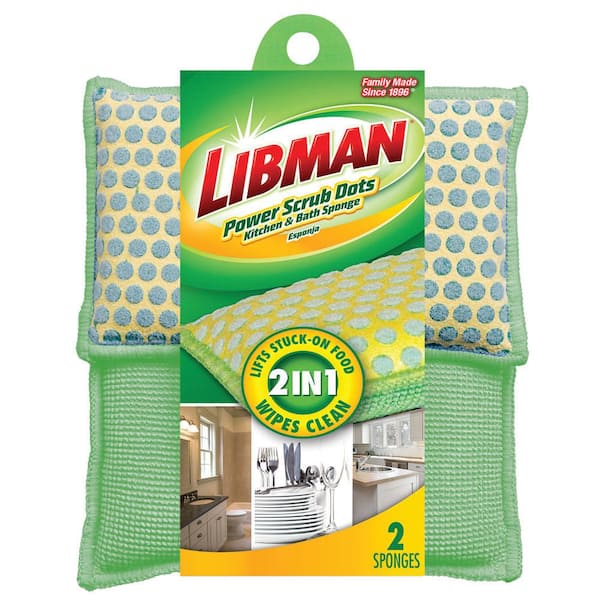The image features a packaged Libman Power Scrub Dots Kitchen and Bath Sponge. The rectangular sleeve at the top prominently displays the brand name "Libman" in red, with "Power Scrub Dots" underneath in green, followed by "kitchen and bath sponge" and a Spanish word. The packaging is designed for retail display with a hook at the top. On the front, it states "family made since 1896" and highlights that these sponges "lift stuck on food" and "wipe clean". The packaging also emphasizes the "two-in-one" functionality of the product. Towards the bottom right, there's a yellow section indicating that the package contains two sponges. The packaging features three images: clean plates and silverware in the center, a bathroom on the left, and a kitchen on the right. Within the package, the top sponge is yellowish with blue dots and a green outline, while the bottom sponge is predominantly green with white stripes, showcasing a textured and effective cleaning surface.